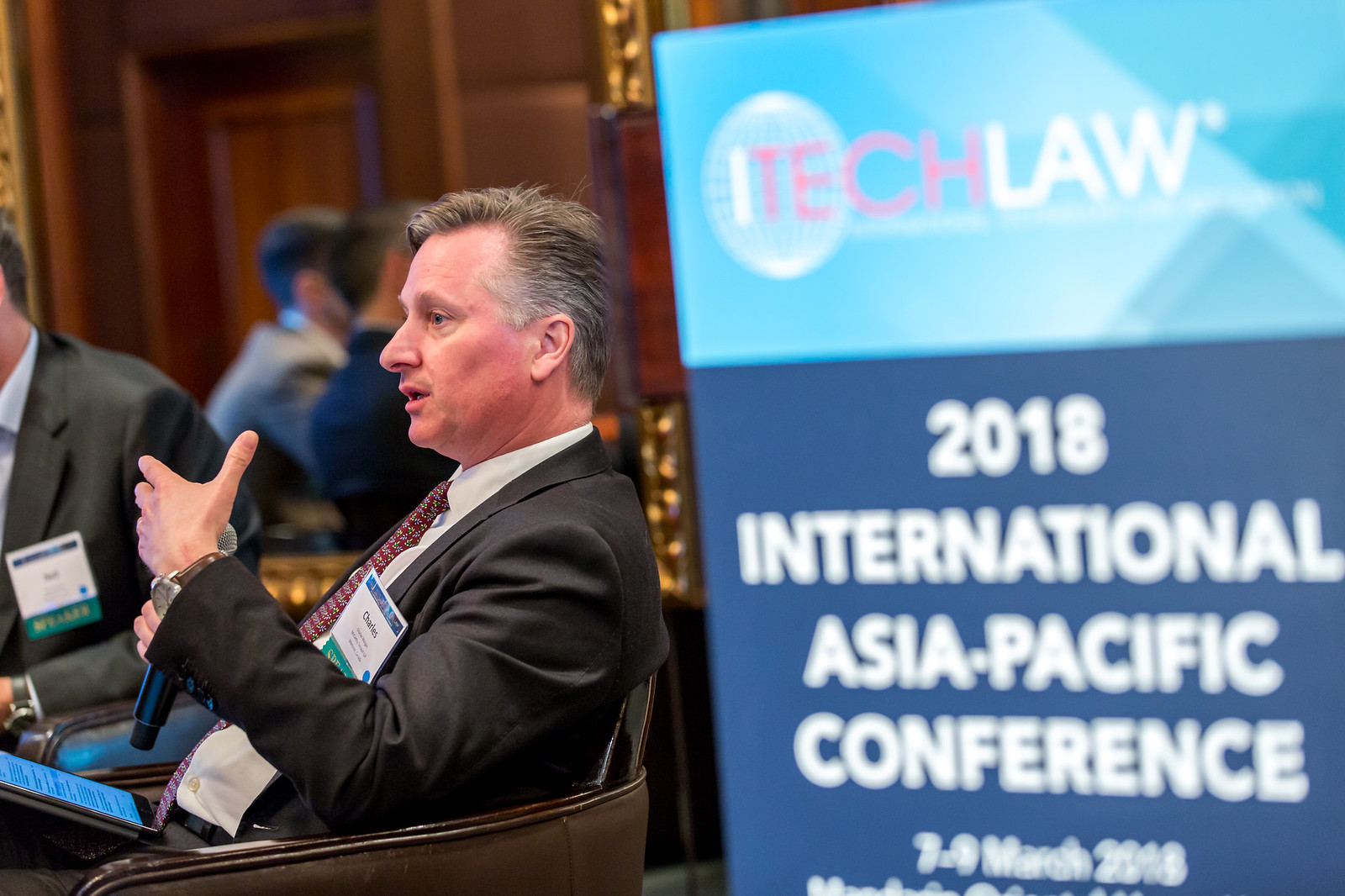In this photograph, a middle-aged man, likely in his 40s or 50s, is seated in a brown chair, facing to the viewer's left. He dons a dark gray suit with a white shirt and a red tie adorned with designs. His appearance is marked by his slicked-back gray and brown hair. He holds a microphone in his right hand and seems engaged in explaining something. Resting on his lap is a digital tablet. The setting appears to be a conference, as indicated by a prominently displayed sign that reads, "iTech Law 2018 International Asia-Pacific Conference," with the dates 7-9 March 2018. The sign features 'Tech' in pink letters on a blue background and 'Law' in white on a darker blue background, all framed in a wooden, gold-accented frame. Surrounding the main speaker are several other individuals also dressed in suits; however, their faces are either partially obscured or out of the frame. The room itself has brown wooden elements, enhancing the formal ambiance of the conference.